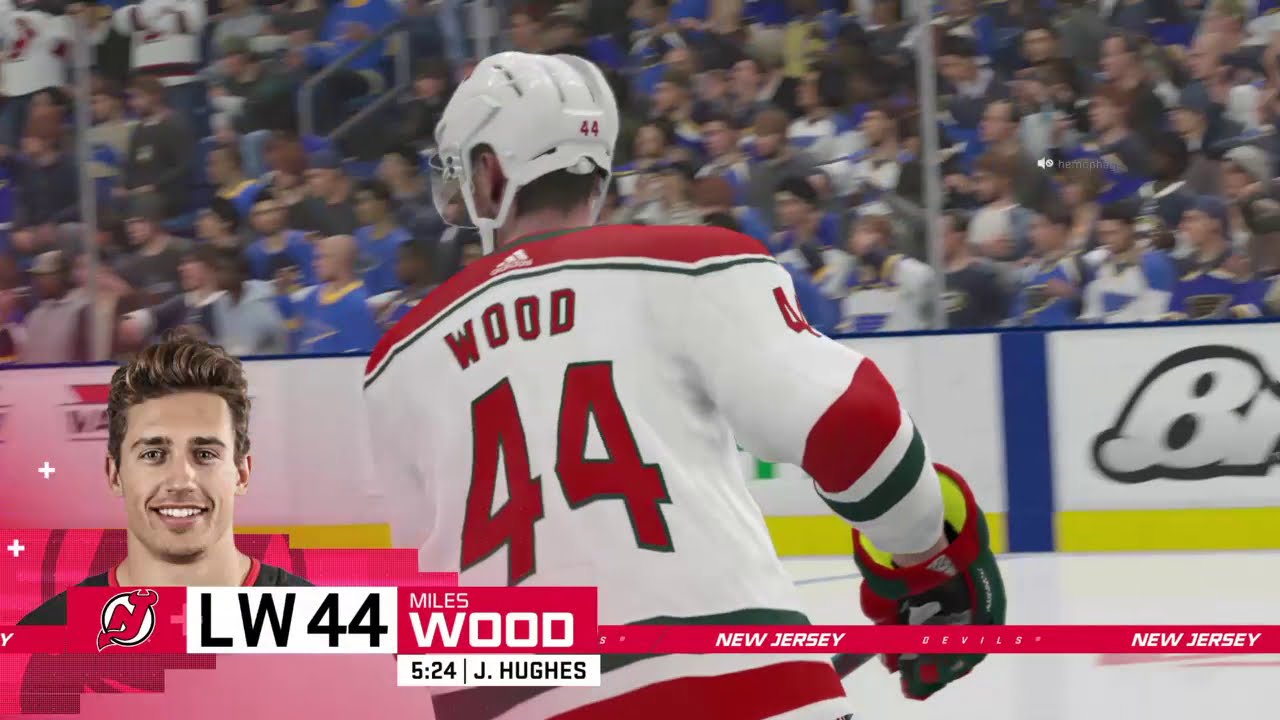The image showcases a highly detailed NHL hockey video game featuring Miles Wood of the New Jersey Devils. The main focus is on Wood, who is depicted from the back with his jersey number "44" and last name clearly visible in red on a predominately white uniform, accented with green. His white helmet gleams under the lights, capturing the realism of the game’s graphics. Positioned slightly off-center to the left, the virtual Miles Wood appears to be skating, with his gaze directed towards the action on the ice. 

In the bottom left corner of the image, there's a headshot of the real-life Miles Wood, smiling and showing off his brown hair. The infographic beneath this headshot reads “Left Wing 44 Miles Wood” and “New Jersey Devils, New Jersey.” 

The background of the image features an array of digital hockey fans, predominantly decked out in St. Louis Blues jerseys of blue and yellow, adding to the immersive game environment. The blurred crowd gives a sense of dynamic movement and excitement. The arena boards showcase various sponsors, including the EA Sports logo, while the ice reflects the intense, competitive setting of an NHL game. The visual composition and level of detail in this video game capture the lively atmosphere of a real-life hockey match.